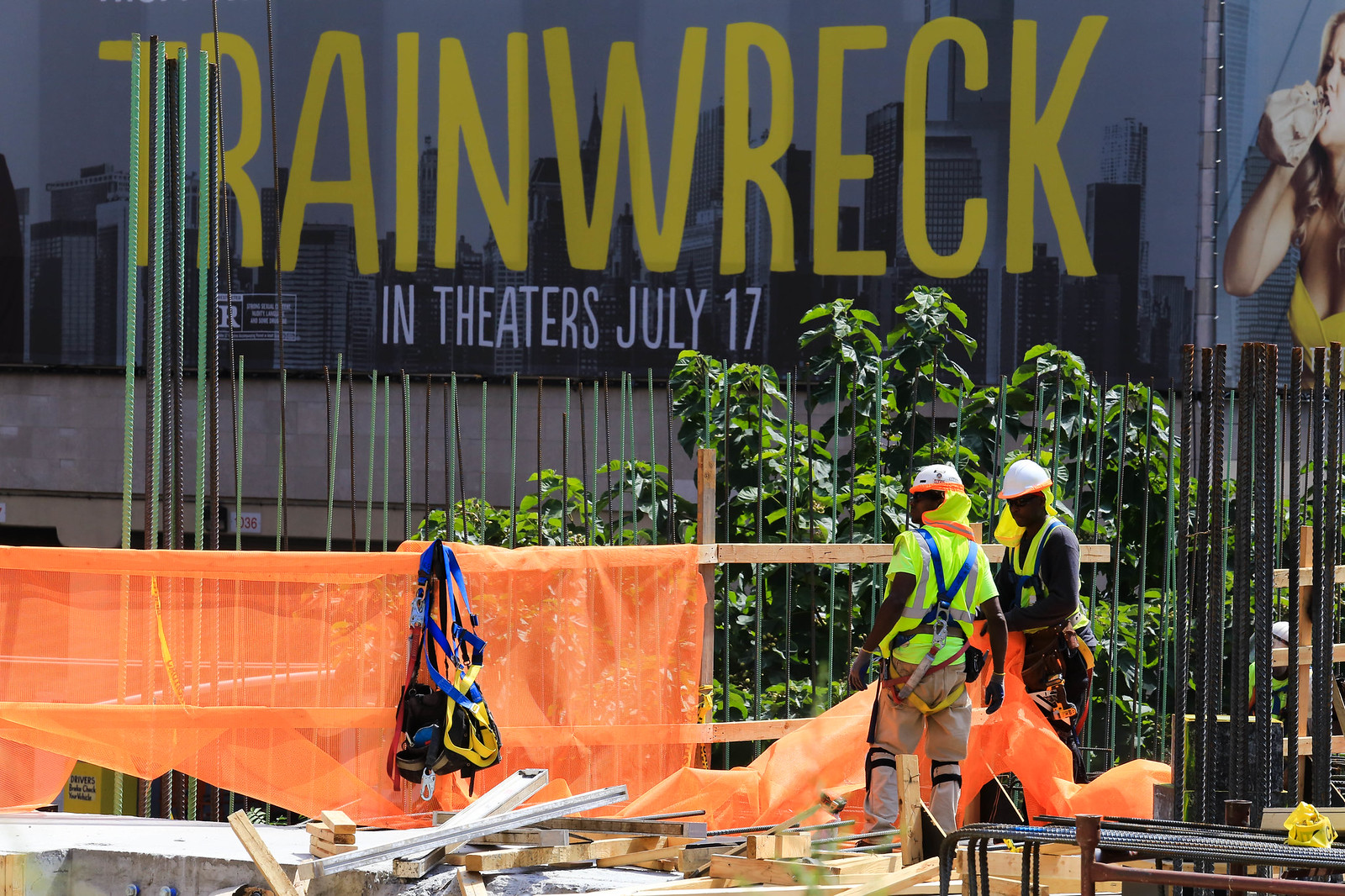In this outdoor color photograph, two dark-skinned construction workers, both wearing white hard hats and yellow high-visibility safety vests, are actively engaged in construction work. The worker on the left wears a neon yellow short-sleeved t-shirt, while the one on the right sports a black long-sleeved shirt underneath his safety vest. They are seen installing wooden beams and attaching sheets of bright orange plastic mesh to the framework. Pieces of wood and metal rebar are scattered around the foreground, alongside what appears to be a low stone wall and various plant life. Dominating the background is a sleek, black glass building adorned with a prominent sign. In large yellow capital letters, the sign reads "TRAINWRECK," with smaller white text below stating "IN THEATERS, July 17th," complete with an R-rating emblem from the Motion Picture Association. At the far right of the image, a female figure clad in yellow is drinking from a container wrapped in a paper bag, subtly contributing to the bustling scene.